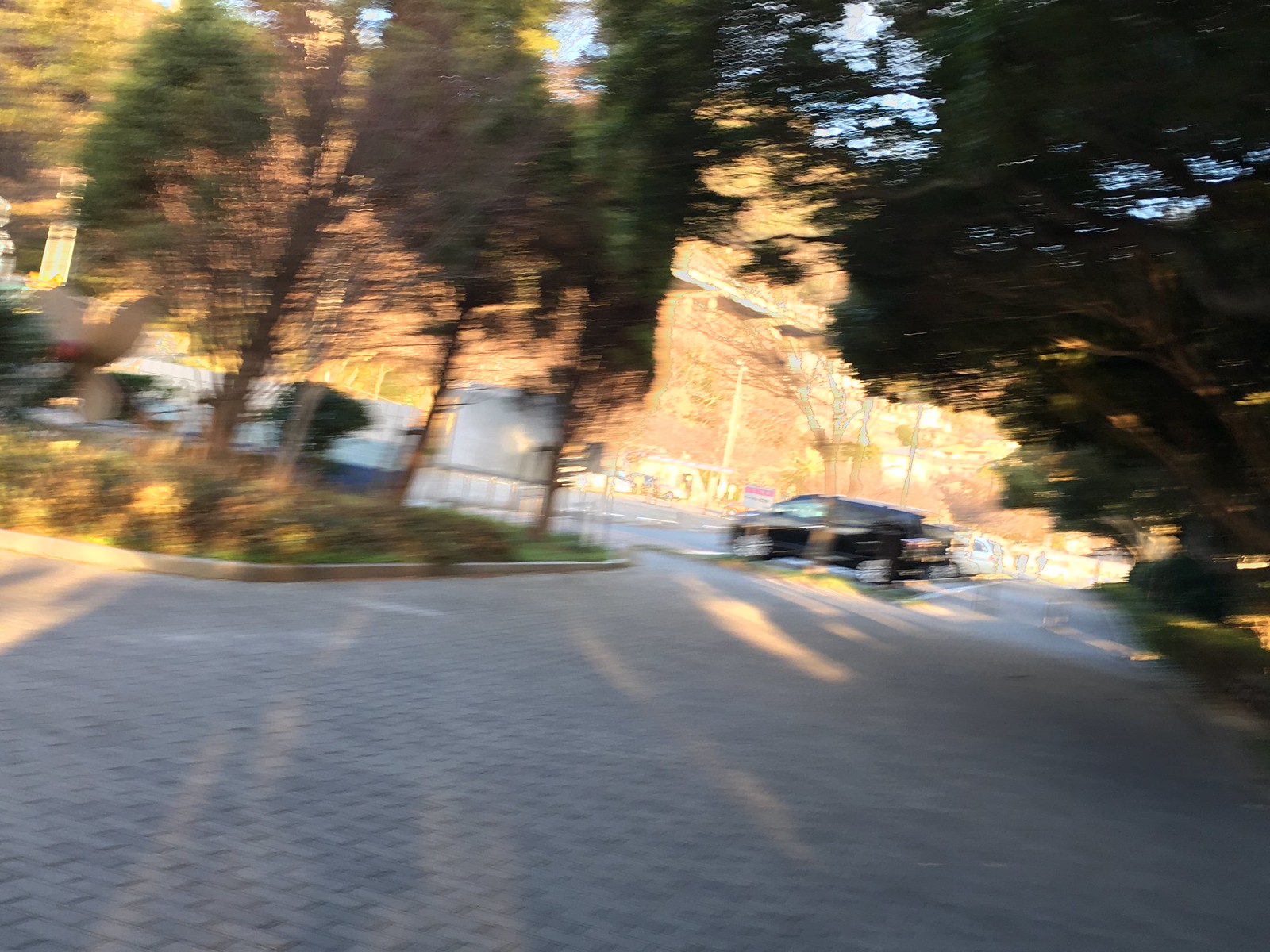A slightly blurred, angled photograph captures a grove of small trees and shrubs with the potential for further growth. The lot they are situated in contains what appear to be brownish bricks, though their exact color is difficult to discern due to shadows cast across the scene. In the background, a dark-colored van or SUV is partially visible in a blurred parking lot, alongside what might be another vehicle, possibly white in color, though its details remain obscure. The image was taken during daylight hours, as evidenced by the sun casting a distinct glare and shadows over the entire scene.